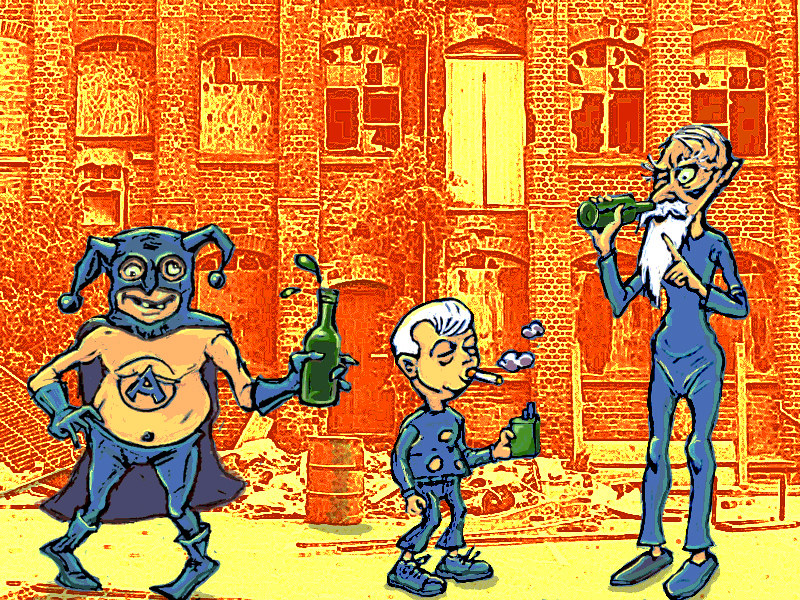In this cartoon artwork, three eccentric cartoon characters stand against the backdrop of a dilapidated red brick building with broken windows, washed in a bright orange-yellow hue. The first character on the left is a disheveled, drunken man dressed in a blue jester-like costume with a cape, blue gloves, tights, and boots. He has a cowl with ear-like protrusions, no shirt, and an “A” symbol within a circle on his chest. His eyes point in different directions, and he is missing several teeth, holding a green bottle in his hand. In the center, there's a short old man characterized by his blue, tattered clothes which include a holey long-sleeve shirt, exposed ankles, and blue shoes. He has white-gray hair and smokes a cigarette, clutching a green pack of cigarettes in his left hand. To the right, the tallest character is an emaciated old man with a long white beard, thinning hair, and wild eyebrows. Dressed entirely in blue clothes that resemble a bodysuit and blue slippers, he is swigging from another green bottle, raising a finger, and fixing an intense gaze with one eye closed. All three appear to be old, Caucasian men engaged in vices, hinting at a somber commentary on life's potential pitfalls.